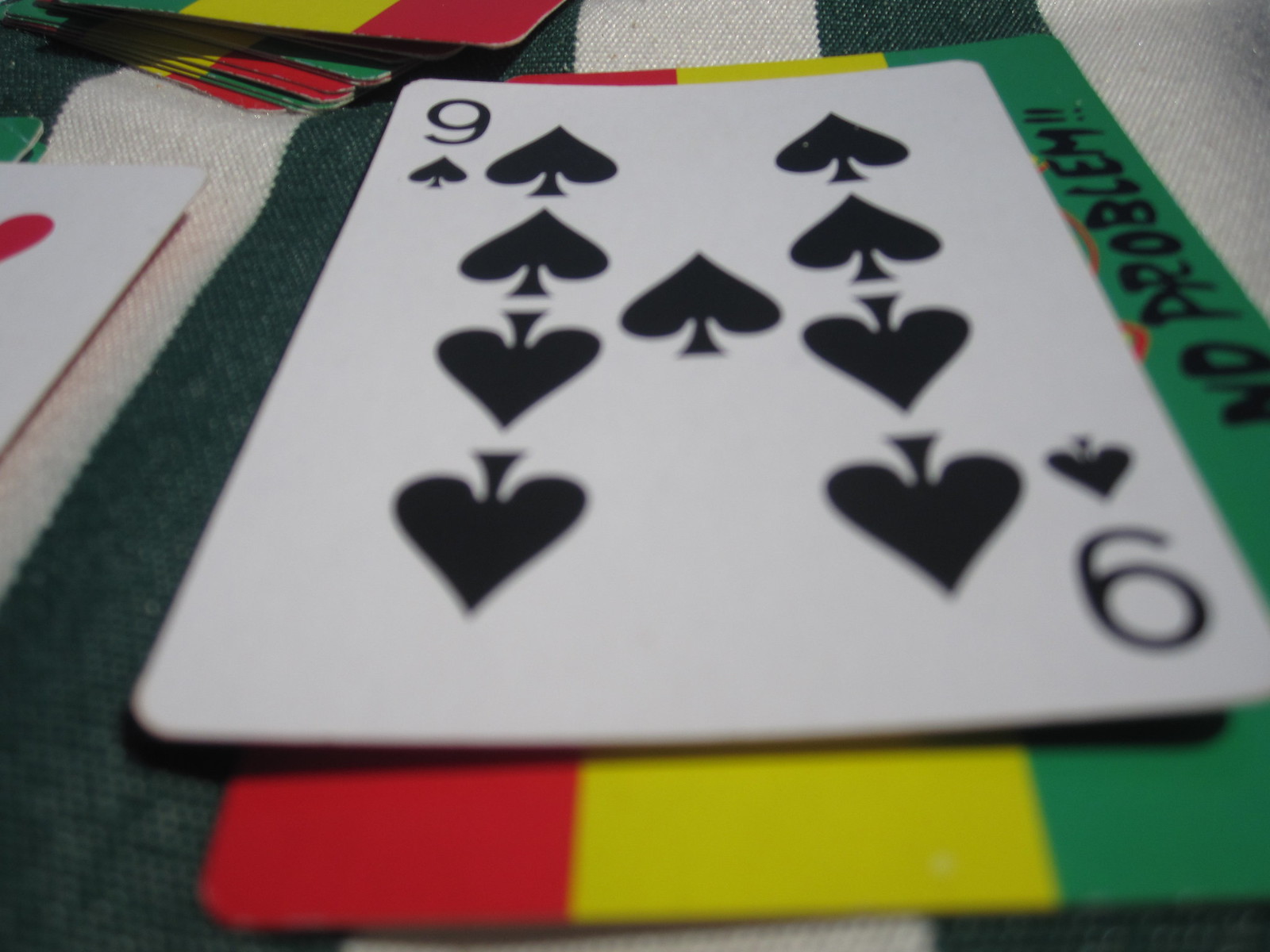This detailed close-up photograph showcases a playing card with a focus on its intricate design elements. The foreground of the image is artistically blurred, drawing attention to the clear and sharp background. To the left of the main card, a partial card can be seen, accompanied by a stack of upside-down cards situated at the top left corner of the frame. All cards rest on a textured dark green and cream blanket adorned with vertical stripes. 

The playing cards feature traditional faces on one side, while the reverse side displays a vibrant design of vertical stripes in red, yellow, and green. A distinctive element of the design is the bold black font reading "No Problem," which runs vertically within the green stripe on the border. 

The card that is fully visible and in focus is the nine of spades. The two nines are located in the top left and bottom right corners, although the bottom right corner is slightly blurred. The nine spades are arranged in a column, aligning vertically with a single spade positioned in the center of the card. The overall composition of the photo combines a mix of clarity and blur to create an intriguing visual experience.